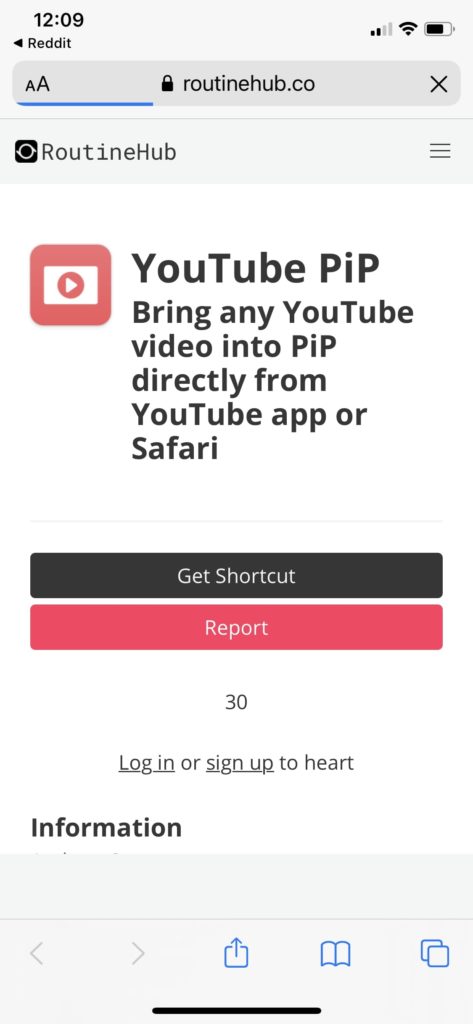This is a detailed screenshot of a smartphone interface. The background consists of gray and black gradients. The current time, displayed on the left-hand side, reads 12:09.

Below the time, a black triangular icon pointing left is displayed, next to which the word "Reddit" appears in black text. Following this, a browser interface is visible, characterized by a gray rectangular shape. On the left side of the browser's address bar, there is a small uppercase 'A' next to a slightly larger uppercase 'A', accompanied by a black padlock icon. The browser address bar shows the URL "RoutineHub.co" in black text and includes a black 'X' icon for closing the page. 

The loading process of the page is indicated by a thin, partially completed blue line underneath the address bar. Below this, there is a thin gray line stretched across the screen.

In the main section of the screenshot, a black square is seen with a white circle at its center, labeled "RoutineHub." To its right, three black horizontal lines are present, suggesting a menu icon.

The remaining space is predominantly white, centered by a prominent red square containing the YouTube logo: a white rectangle within which is a red circle housing a white triangle. This emblematic logo is captioned "YouTube PIP" in black text, followed by the description, "Bring any YouTube video into PIP directly from the YouTube app for Safari." This indicates a feature related to Picture-in-Picture (PIP) playback.

Below this, another thin gray line extends across the width of the screen, followed by two adjacent buttons. The first button is dark gray with white text reading "Get Shortcut," while the second is red with white text stating "Report."

Further down, there is some additional text in black, indicating the number "30" and an instruction to "Log In or Sign Up to" complete or access additional features.